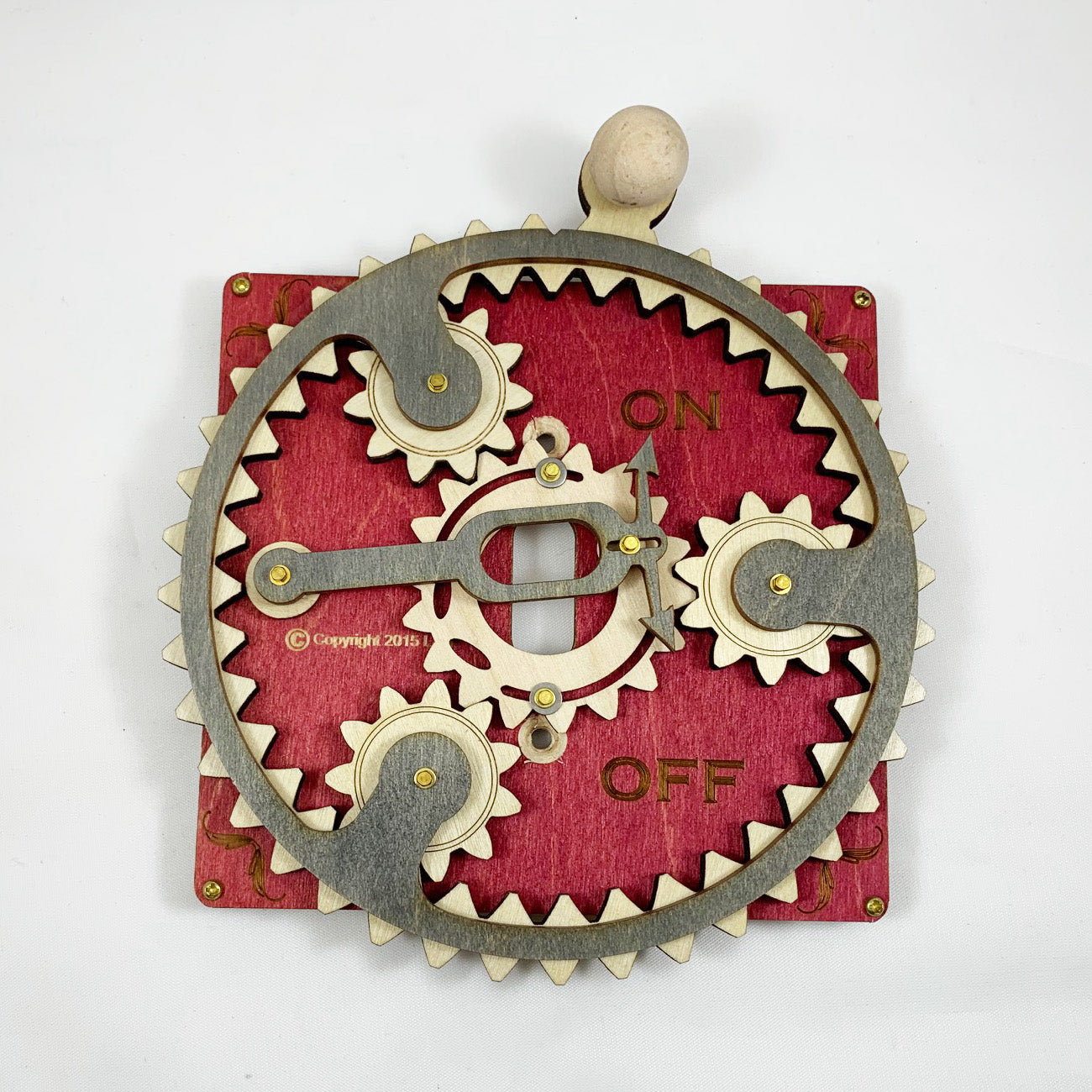This photograph features an intricate arrangement of interconnected gears set against a red square wooden background. Dominating the visual is a large circular formation made up of multiple gears, with three prominent tan gears extending towards the center, all interlocking with a larger central gear. This central gear appears to function as a switch, capable of toggling between positions marked "ON" and "OFF" depending on the direction in which the gears are turned. A lever extends from the left towards the middle, flanked by arrows pointing towards the "ON" and "OFF" markings, effectively indicating the active position of the gears. The words "ON" and "OFF" are inscribed in golden brown letters on the top right and bottom right of the wooden surface respectively, and the background has a warm red hue. Adding to the detailed design, the central portion of the composition is marked by smaller gears and clock arrows, suggesting a timepiece-like mechanism. The intricate setup is accentuated by elements of triangular teeth-like protrusions and a small embossed text on the middle left reading "copyright 2015".